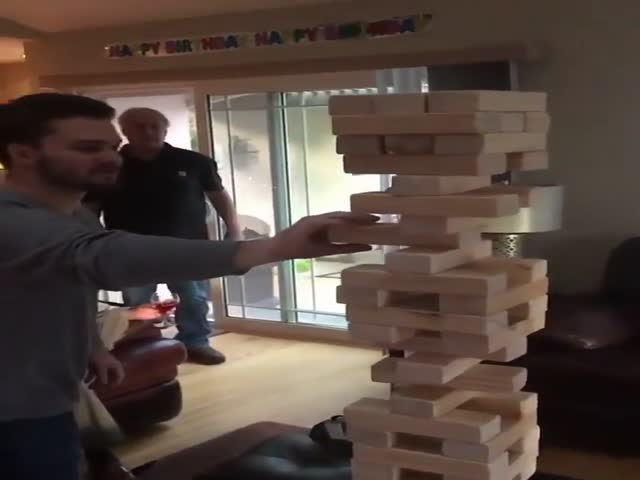In the photograph, the left side captures a partial view of a white man with dark hair, a beard, and a mustache. Despite the dim lighting, his gray shirt is visible as he extends his right hand toward a precariously stacked tower of plywood pieces, evidently participating in a game where the goal appears to be removing a plank from the midsection without causing the structure to collapse. In the background, another man, likely in his 50s, is seen. He is also a white man, heavyset, attired in a dark polo shirt and blue jeans. Behind him is a glass door that seemingly leads to a patio. The image is completed by a light brown hardwood floor underfoot.